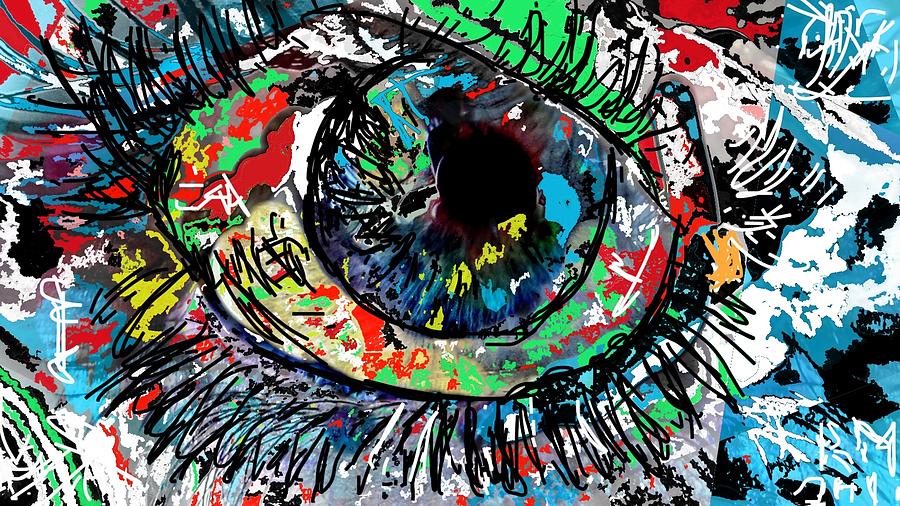This vibrant and dynamic artwork features a prominently detailed eye as its focal point, meticulously rendered with an array of striking colors. The pupil is a jet black circle situated at the center, surrounded by an iris that blends greens, blues, and yellows, intricately highlighted with black streaks. The eye itself is framed by thick black lines, accentuating the long, expressive eyelashes that extend above and below the eye.

The surrounding area of the eye is a chaotic yet captivating explosion of colors: reds, blues, whites, greens, and yellows, all splashed irregularly across the canvas. On the right side of the image, hues of blue, white, and black dominate, with splashes of red and yellow towards the top. The left side, in contrast, showcases more reds and medium blues, with touches of black, white, and green.

Overall, the painting exudes an intense, almost furrowed emotion, enhanced by the eye's vivid detail and the abstract, energetic paint splatters that envelop it, creating a unique and captivating visual experience.